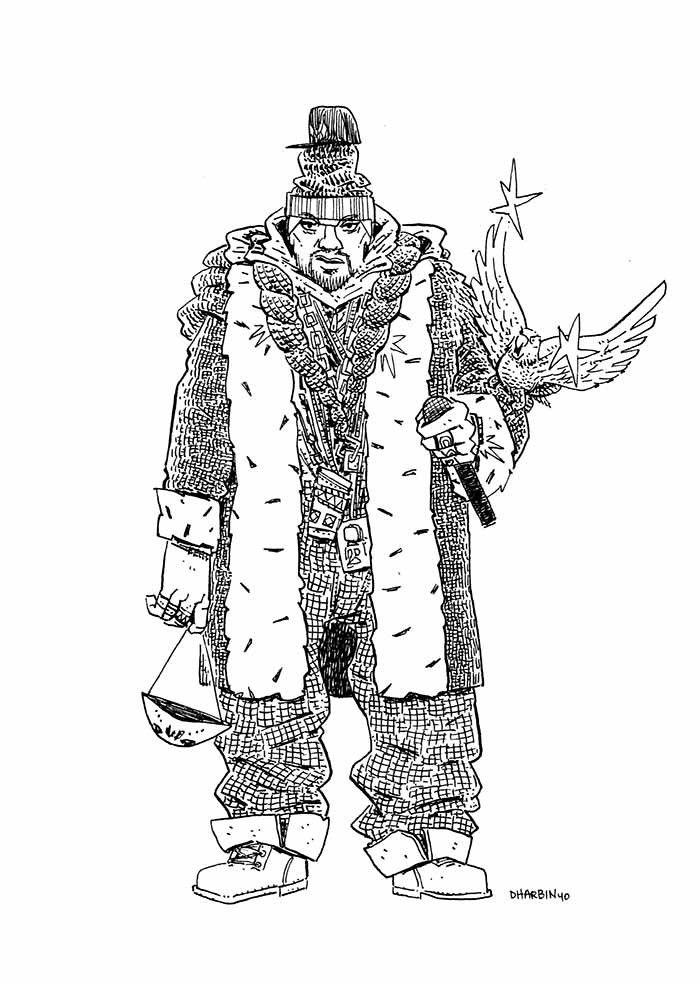In a detailed pen sketch, the renowned figure of Ghostface Killah from the Wu-Tang Clan is depicted with various intricate elements. The character is holding an old hockey mask in his right hand, dangling by a string from one finger. His left hand clutches a cordless microphone, adorned with multiple rings. A bird with outstretched wings and stars is prominently inked on his left forearm. The ensemble includes a snug stocking cap topped with a baseball cap, a goatee, and a stern expression sketched on his face. Ghostface is dressed in an oversized padded coat featuring a large furry collar, layered with numerous chains and plaques around his chest and neck. Plaid pants, which are bunched up and turned at the cuffs, and laced Timberland-like boots with tongues flapping over the sides complete his outfit. The entire image remains unpublished in the comic world, uniquely capturing Ghostface Killah’s iconic rap persona.